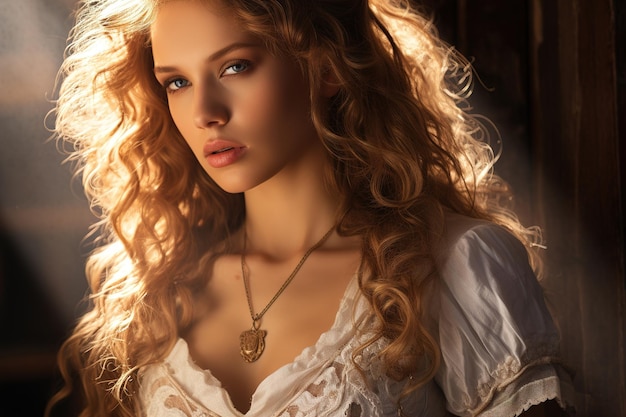The image captures a striking and detailed portrait of a young blonde-haired Caucasian female with very long, curly hair that cascades halfway down her back and over her shoulder. Her blue-gray eyes and very full, lush lips—with a hint of red—add to her vibrant appearance. She wears a gold-colored pendant necklace and a delicate, white lacy short-sleeved top. The photograph, presented in a square format, shows her from just below her breasts to the top of her head, leaving the rest of her outfit undisclosed. It is set indoors with sunlight streaming diagonally in from the upper left corner, creating a stark contrast with the dark right side of the image. The light highlights her features, casting part of her face in shadow, and there's no discernible background except for what appears to be a paneled wall. The overall effect is a beautifully lit portrait that emphasizes her natural beauty.